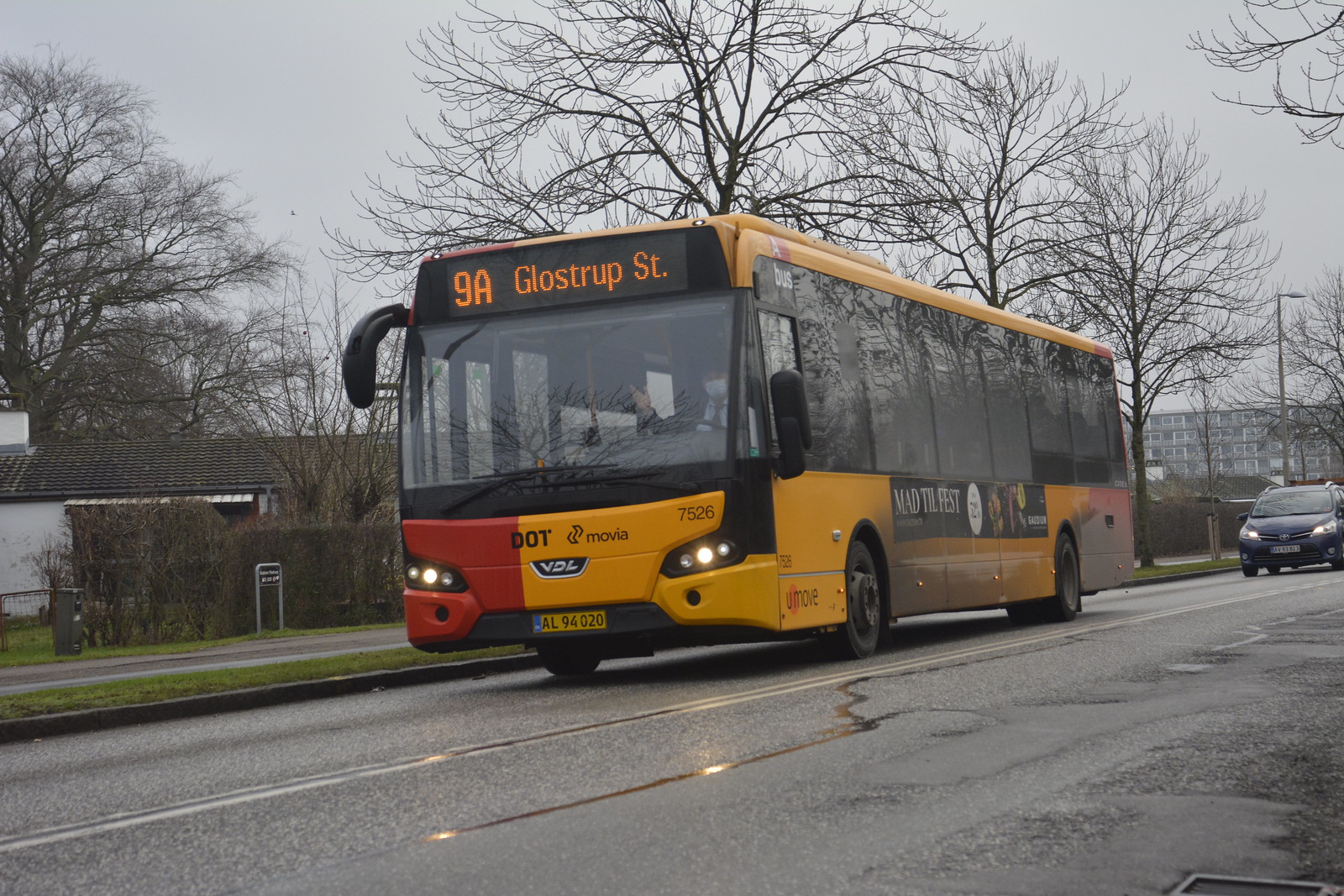This is a rectangular photograph taken outside on a gloomy, overcast day, likely during late winter or early spring, as indicated by the bare branches of the tall trees framing the scene. The sky is a uniform gray, hinting at recent rain which has left the asphalt street looking damp. In the background, a large apartment building looms, featuring double-doored windows leading to patios. 

On the left side of the image, there are residential buildings with gray rooftops, bordered by shrubs and a grassy median. Moving towards the center-right, the image captures a vibrant yellow city bus, distinguished by its red front bumper and large windows with black frames. The bus is in motion, heading to the left, with illuminated signage reading "9A Galstrop Street" at the top. The left side of the bus features an advertisement that reads "Mad Till Fest," set against a red and yellow backdrop.

A blue car, headlights piercing the dim light, follows closely behind the bus. The bus driver, visible through the tall windshield, is wearing a tie and a face mask. The street is marked with a double yellow line and is flanked by a sidewalk and a hedge. A lone streetlight stands guard, illuminating the damp scene.